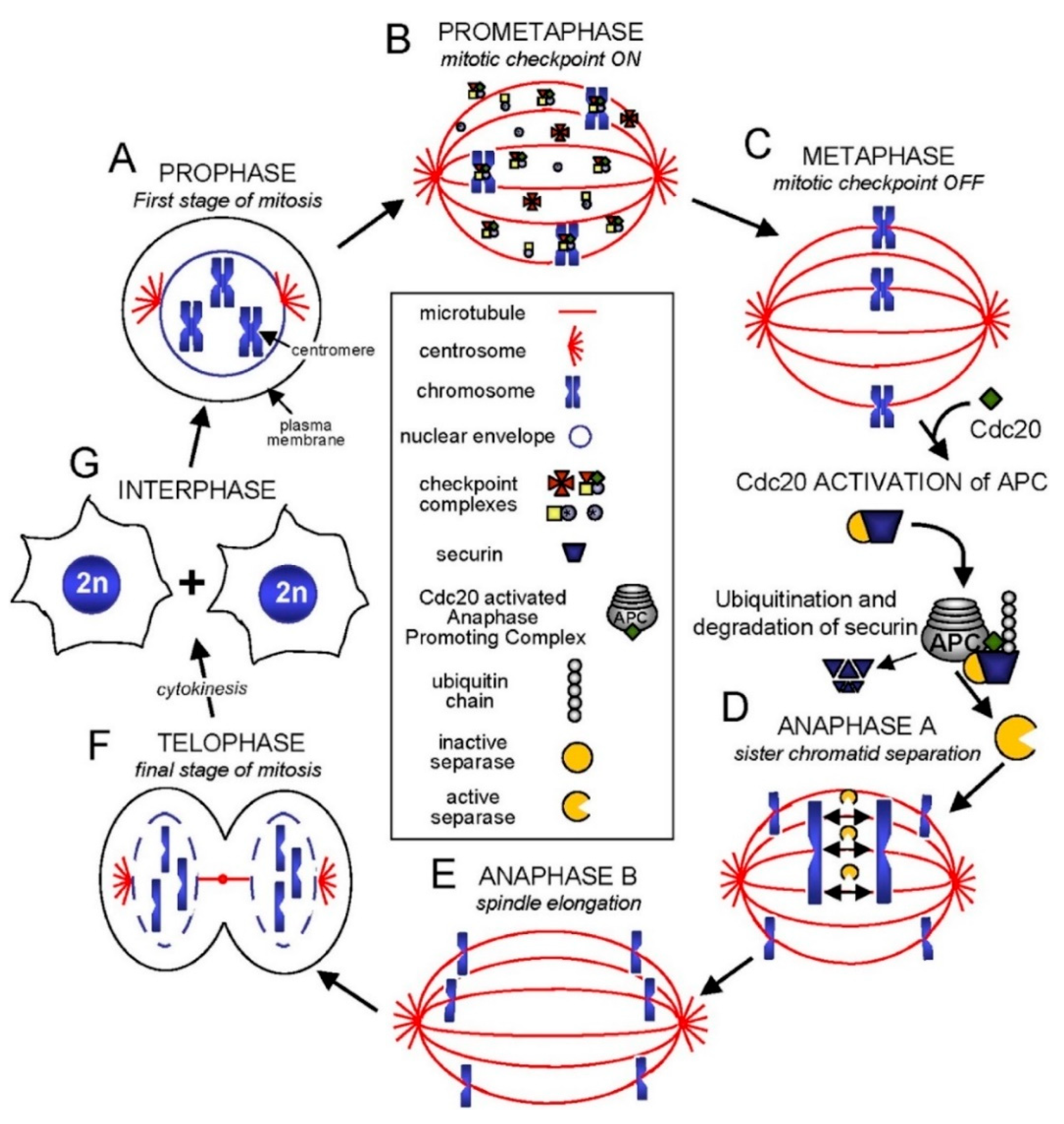The image is a detailed, hand-drawn infographic on a white background, illustrating the stages of the cell cycle, specifically mitosis. The cycle is depicted in a circular flow chart divided into eight labeled sections (A through H), each representing different stages and processes of mitosis. 

1. **Prophase (A)** - This is the first stage, showing a circle with three blue X's representing chromosomes.
   
2. **Prometaphase (B)** - Indicates the mitotic checkpoint is on, ensuring the cell is ready to proceed with mitosis. This section features a red circle with lines and black crosses.

3. **Metaphase (C)** - At this stage, the mitotic checkpoint is off, and chromosomes are lined up in the middle of the cell. The red circle with three blue X's shifting downward is depicted here.

4. **Anaphase A** - Highlights the ubiquination and degradation of securin, depicted by a bottle-like illustration with blue cups.

5. **Anaphase B (D & E)** - Shows spindle elongation with a red circle and arrows, representing the movement of chromosomes.

6. **Telophase (F)** - The final stage of mitosis, illustrated with a circle featuring blue lines.

7. **Interphase (G)** - Depicted with two blue-centered, fried egg-like images labeled with "2n", representing the period when the cell is not actively dividing.

8. **Summary in Center** - The middle of the diagram provides a legend explaining the icons: blue X's for chromosomes, black crosses for microtubules, and cup-like shapes for inactive securin.

The circular flow captures the repetitive nature of the cell cycle, emphasizing the critical stages and various structural components involved, like the chromosome, nuclear envelope, centrosome, and their interactions.